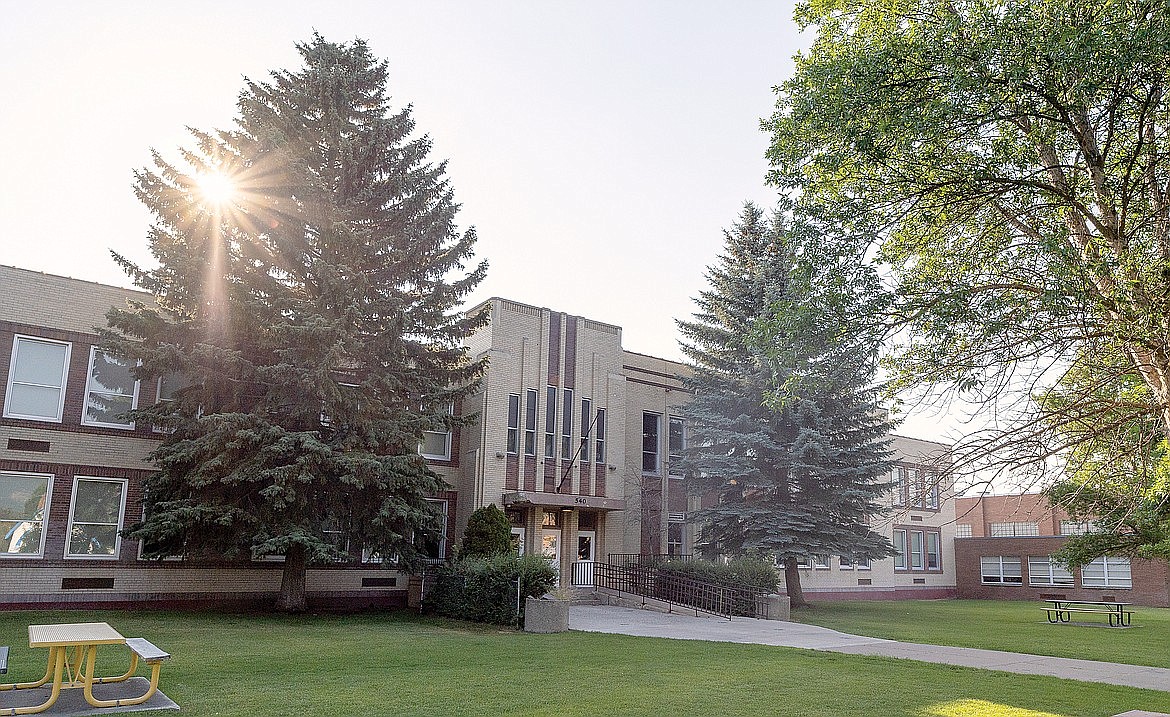The image depicts the front of a modern university building, characterized by its gray and red brick facade. The building features three large entrance doors centrally located and flanked by substantial windows. The scene, captured on a bright, sunny day with a clear blue sky, is framed by two tall evergreen trees. The vibrant green lawn in front is well-maintained, with a concrete ramp for wheelchair access and a set of stairs to the left.

Adjacent to the entrance, on both the left and right sides of the image, are picnic tables. The table on the left is distinctly yellow, while the color of the table on the right is less discernible but appears darker. Additionally, a tall green tree partially shades the area, diffusing the sunlight and providing a clear view of the setting without glare. The overall ambiance suggests an inviting space within a lush, well-kept natural environment, ideal for a college campus. The presence of additional trees, one more evergreen and another with green leaves, further enhances the scenic beauty of the photograph.